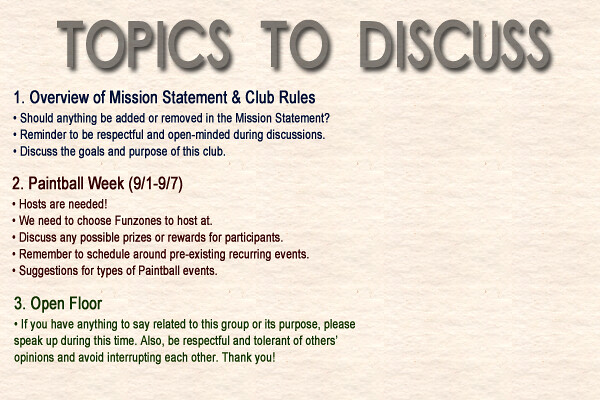The image displays a PowerPoint slide with a textured white paper background. The heading "Topics to Discuss" is written in dark grey text and features a drop shadow effect. Below the heading, the content is organized into three main sections with numbered bullet points, each presented in different colors.

1. **Overview of Mission Statement and Club Rules** (dark blue text)
   - Should anything be added or removed in the mission statement?
   - Reminder to be respectful and open-minded during discussions.
   - Discuss the goals and purpose of this club.

2. **Paintball Week (September 1st to September 7th)** (dark red text)
   - Hosts are needed.
   - We need to choose fun zones to host at.
   - Discuss any possible prizes or rewards for participants.
   - Remember to schedule around pre-existing recurring events.
   - Suggestions for types of paintball events.

3. **Open Floor** (dark green text)
   - If you have anything to say related to this group or its purpose, please speak up during this time. Also, be respectful and tolerant of others' opinions, and avoid interrupting each other. Thank you.